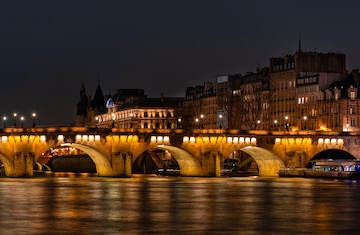This is a serene and captivating nighttime photograph of a cityscape featuring a low, arch-based bridge illuminated by lights along its arches and edges. The foreground presents a calm body of water reflecting the lights from the bridge and surrounding buildings. Behind the bridge, several multi-story buildings, seemingly constructed from brick or stone, rise up, their windows and architectural details subtly visible due to interior lighting. One notable building near the center showcases columns and bright illumination. To the left of the scene, tall, illuminated streetlights stand out. Above the buildings, the sky is pitch black, devoid of the moon or stars, adding to the tranquil beauty of the urban night scene.